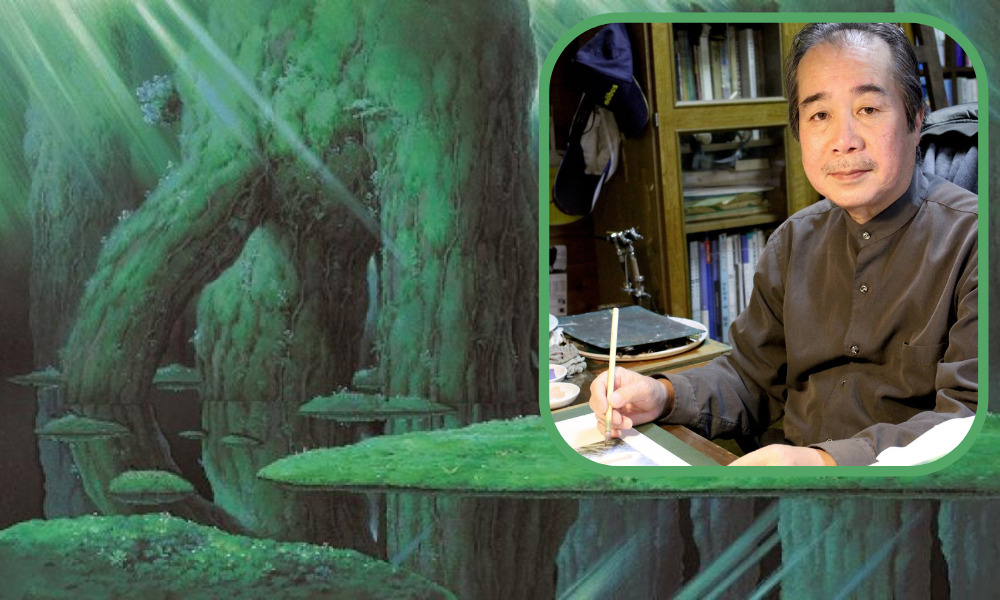The horizontally rectangular image masterfully combines elements of both photography and art. Dominating the right side is a square photograph with a rounded green border, capturing a middle-aged Asian gentleman with a receding hairline and sparse mustache, facing the camera. He wears a fully buttoned gray long-sleeved shirt and holds a pen or pencil in his right hand, seemingly working on a manuscript or piece of paper in front of him. Behind him, books of various sizes fill a shelf, and to the left of the books, there is a witch doll resting on a stack of boxes. 

The left side of the image depicts a fantastical, lush green forest scene with giant tree trunks and floating circles of forest elements such as leaves and grass. Streams of light cascade from the upper left corner, enhancing the ethereal atmosphere. The colors throughout the image range from browns and beiges to various shades of green and blue, creating a seamless blend between the indoor and outdoor worlds. The contrast between the man’s meticulous indoor setting and the vibrant, imaginative forest evokes a sense of juxtaposition between reality and fantasy.